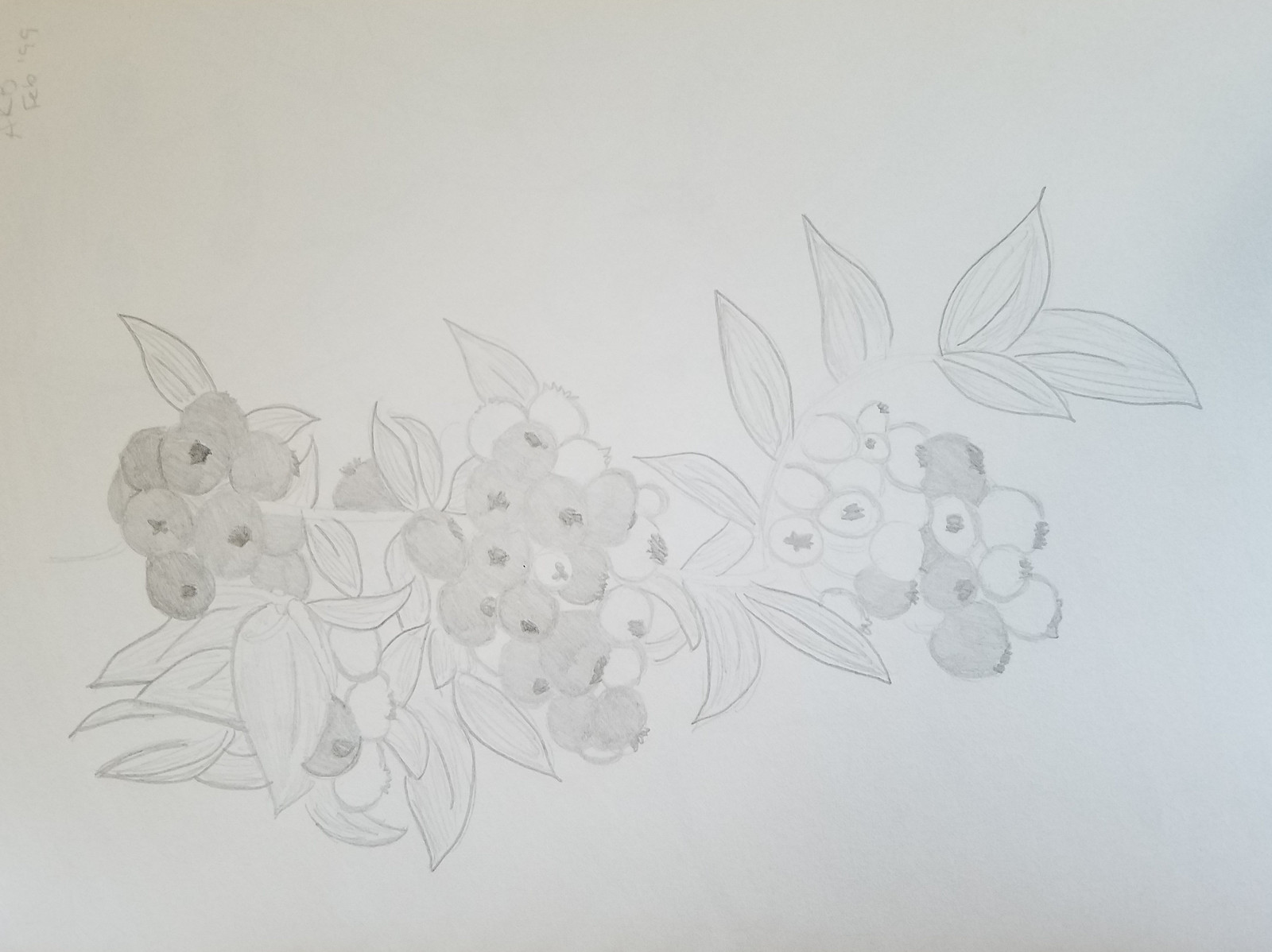This image showcases a detailed pencil drawing on white paper, centered within the frame. The drawing depicts a cluster of small, circular fruits, likely blueberries or grapes, where some are shaded gray with darker centers, while others are left white. Surrounding the fruit are narrow, pointed leaves, each featuring a single vein down the middle. Some of the leaves display subtle pencil shading. Notably, the upper right corner of the white paper includes faint pencil markings. The careful shading and intricate details capture the texture and form of both the berries and leaves, void of an artist's signature. The background of the drawing itself remains gray, adding depth to the artwork.